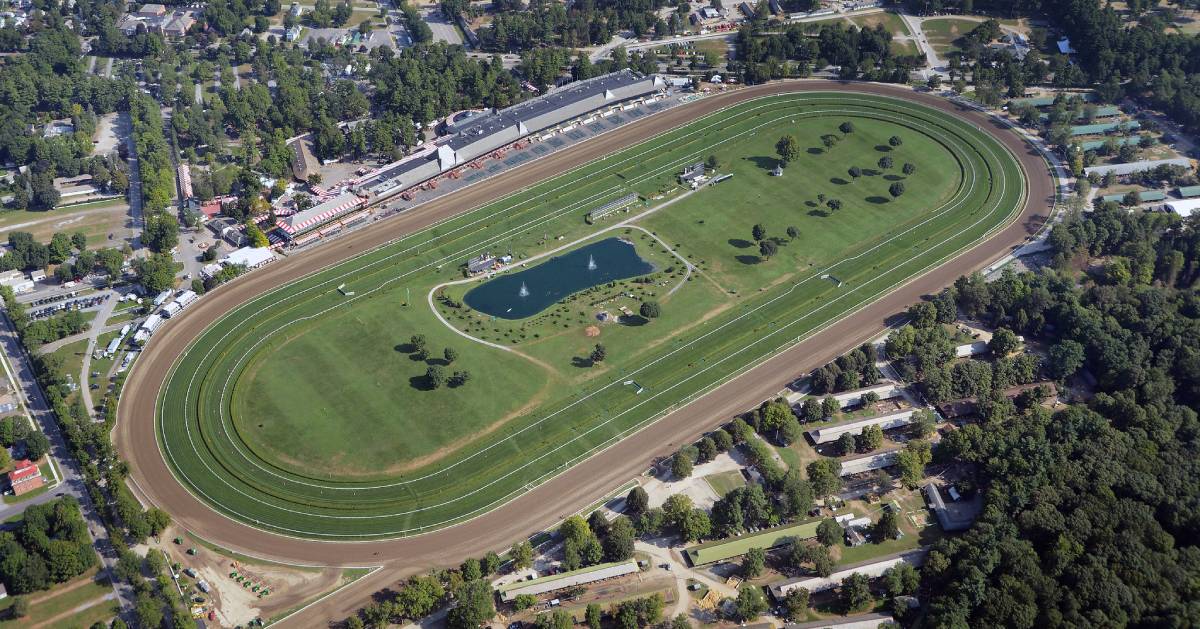The image is a high overhead shot, possibly taken from a plane, helicopter, or drone, capturing a large, oval, pill-shaped track. The track has green grass and a small blue pond situated in the center, resembling a suburban horse racing or derby racing track surrounded by a rich, green setting. The track's outer boundary is a brown pathway, possibly for racing, and is encircled by densely packed homes and greenery, suggesting it might be set in a neighborhood. The top left of the track features a long rectangular building, likely a grandstand for spectators. The surrounding area is dotted with numerous rectangular buildings and lush trees, all under clear daylight, indicating it was taken outdoors with ample natural light.